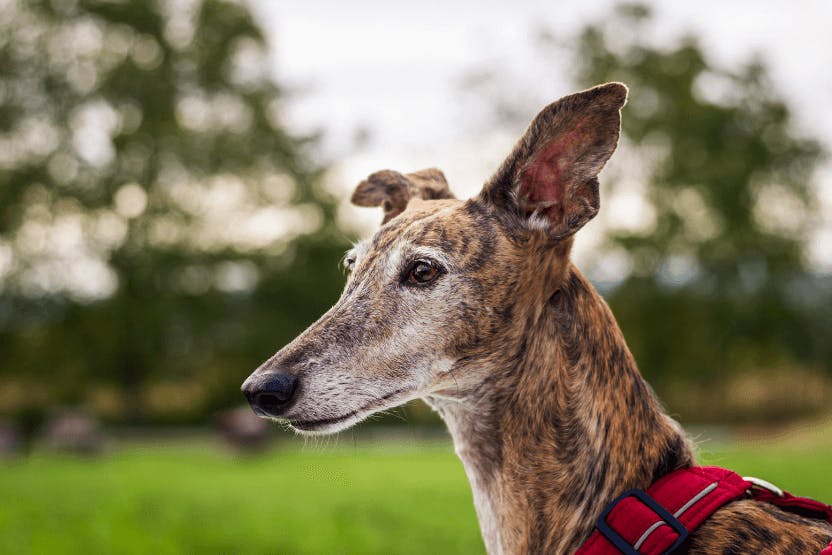This image captures the detailed head and neck of a dog that appears to be a greyhound or a greyhound mix, distinguished by its more pronounced forehead. The dog's long snout and prominent, slightly triangular, pointy ears are notable features, with white accents around the nose and cheeks, and a black nose adding to its distinctive look. The coat showcases a unique, almost striped pattern comprising shades of brown, blonde, and black, creating a speckled effect. The dog wears a visible red harness around its fairly large neck. It is gazing towards the left of the image, set against a blurred background of green grass, vegetation, and trees, suggesting a park-like setting. The depth of field sharply focuses on the dog, accentuating its detailed features amidst a softly obscured background.